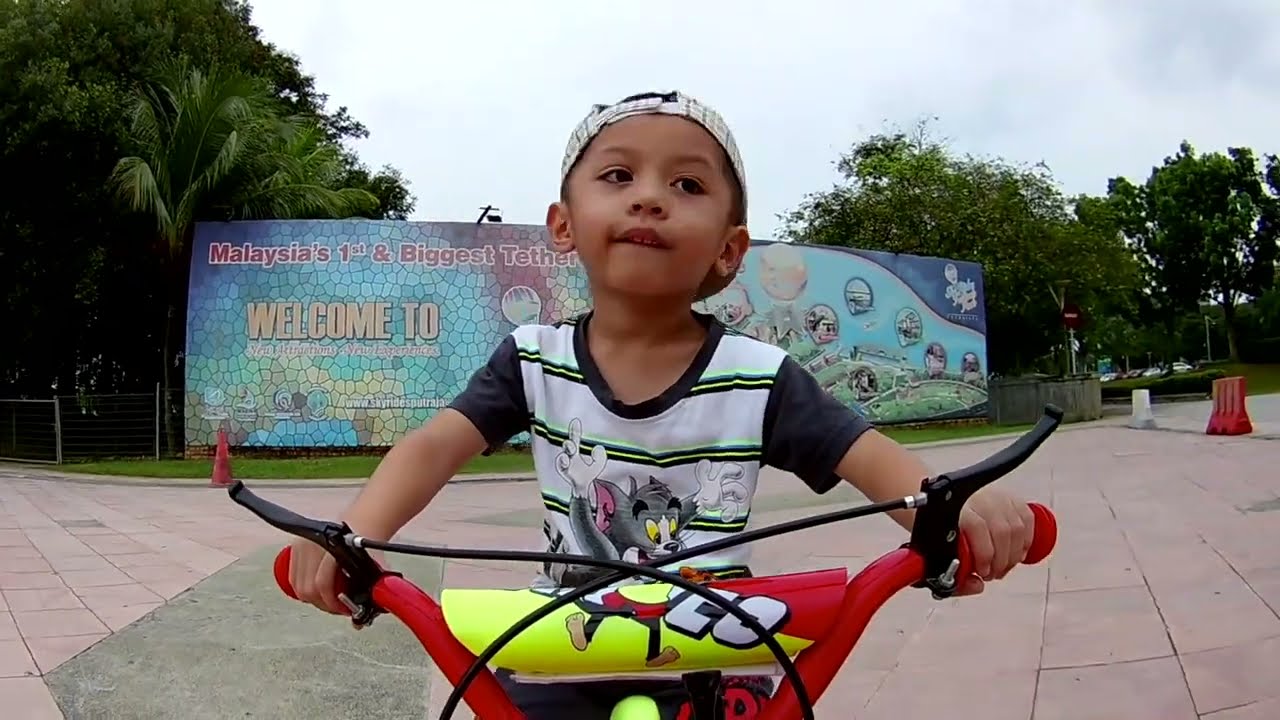This detailed photograph captures a young boy, around three or four years old, riding a red dirt bike or toy bicycle. The boy, who has dark skin, wears a white and black striped baseball cap turned backward. His outfit consists of a white t-shirt with black and yellow horizontal stripes, along with black short sleeves. The shirt features a Tom and Jerry print on the front. The dirt bike itself has a red frame and a padded horizontal bar with a red and yellow cover, which includes a cartoon character and possibly the word "Loco" in white letters. The boy is positioned centrally in the image and is facing the camera, though he appears to be looking slightly to the top left.

The setting is a gray and red pavement sidewalk with some tan-colored stone or concrete tiles visible, indicating a courtyard area. A grassy border surrounds this courtyard. In the background stands a large mural or billboard with a mix of blue, turquoise, dark blue, white, green, and orange colors, featuring the words "Welcome" and "Malaysia's first and biggest tether." However, the remaining text is cut off or illegible. This vividly colorful mural stretches almost the width of the image and sets a lively backdrop for the scene.